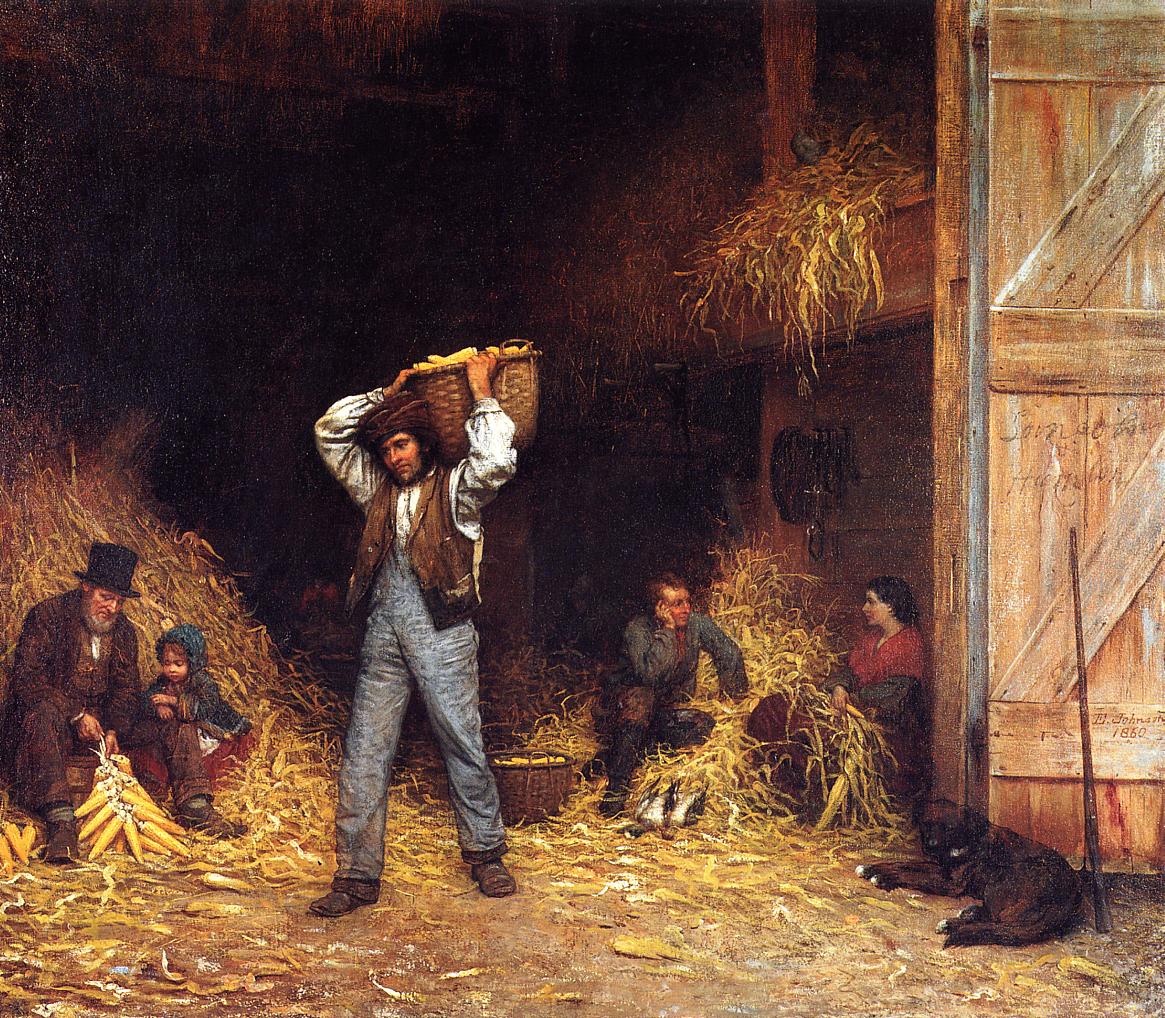This highly detailed and realistic 18th-century-style oil painting depicts a bustling scene inside a rustic barn. Central to the composition is a man wearing a brown vest and gray pants, with brown shoes and a brown head wrap. He is carrying a large wicker basket on his shoulder, laden with produce. To the left, an older man in a black top hat and brown outfit is seated in a pile of hay, husking corn with a small child who is wearing a blue jacket and hooded head covering. The child watches attentively, indicating a moment of quiet instruction.

On the right side of the painting, another man dressed in a blue long-sleeve shirt, brown pants, and boots is engaged in conversation with a woman draped in a red shawl, her brown hair partially covered. They are both comfortably seated in hay. Scattered around them is more hay, two dead birds, and a rifle leaning against the barn door, which is propped open with a stick.

In the foreground, guarding the entrance, sits a brown and black farm dog, adding to the pastoral ambiance. The back of the barn is enveloped in shadow, contrasting with the golden hay spilling out, creating a vivid backdrop. The entire scene is meticulously detailed, from the piles of hay to the distinct textures of the clothing, highlighting the artist's grasp of realism. A faint signature and the date "1860" can be seen on the barn wall, affirming the painting's historical authenticity.